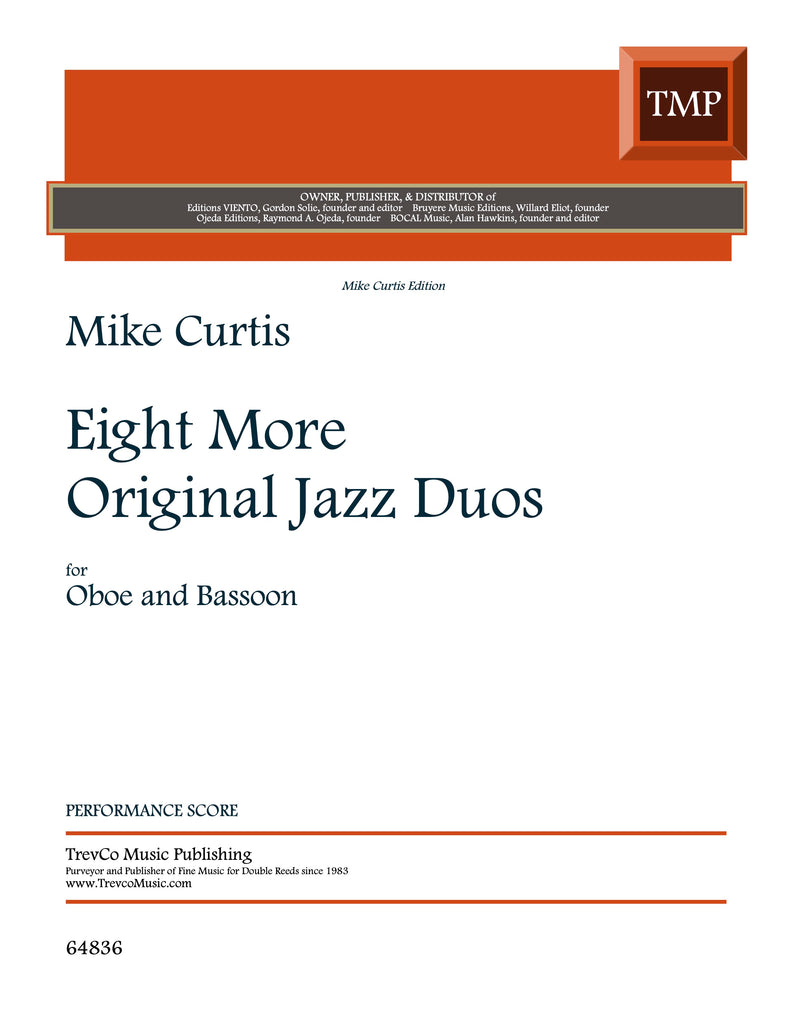The image shows the front cover of a book titled "Eight More Original Jazz Duos for Oboe and Bassoon" by Mike Curtis. The cover features a predominantly white background with text arranged vertically. At the top of the cover, there's a horizontal orange bar with a 3D effect, containing the white letters "TMP" inside a square with red tapered edges on the upper right. Below this bar, a light grey strip with beveled edges houses the text "Owner, Publisher, and Distributor of," followed by the names of various founders and editors, including Gordon Soley, Willard Elliott, and Raymond A. Ojeda. The central part of the cover features the book's title, "Mike Curtis Edition: Eight More Original Jazz Duos," with "for Oboe and Bassoon" and "Performance Score" written underneath in large black text. Towards the bottom of the cover, another thin orange line appears with the text "Trevco Music Publishing," and smaller text underneath reads "Purveyor and Publisher of Fine Music for Double Reeds since 1983." The cover also includes the website "www.trevcomusic.com" and the number "64836."